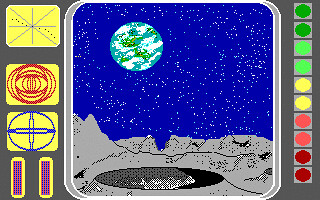A rectangular digital image, possibly from a computer game, depicts a surreal lunar landscape with Earth in the distant background. The scene is framed by interactive gray panel areas on the left and right sides, suggesting that the image may belong to a drawing or design application. These panels contain various buttons and tools used for creating and manipulating the image.

The central view is dominated by a square, bordered by rounded edges. The upper portion of the image features a deep blue expanse speckled with white stars. In the top left corner, Earth is prominently displayed, showcasing greenish-blue hues, swirling white clouds, and visible landmasses.

The bottom half of the image is characterized by the moon's surface, rendered in a slightly rocky gray texture. A dark-centered crater marks the center of the lunar landscape.

On the right gray strip, a vertical array of color circles is displayed. The top two circles are green, followed by two lime green circles, then two yellow circles, two reddish-pink circles, and finally, two burgundy-red circles. These circles appear to be color selection tools for drawing.

The left panel contains three vertical yellow rectangles, each featuring different shapes. The middle rectangle displays a series of red circles, while the one below contains a blue circle with a cross in its center. These shapes seem to serve as drawing aids for creating or enhancing the digital artwork.